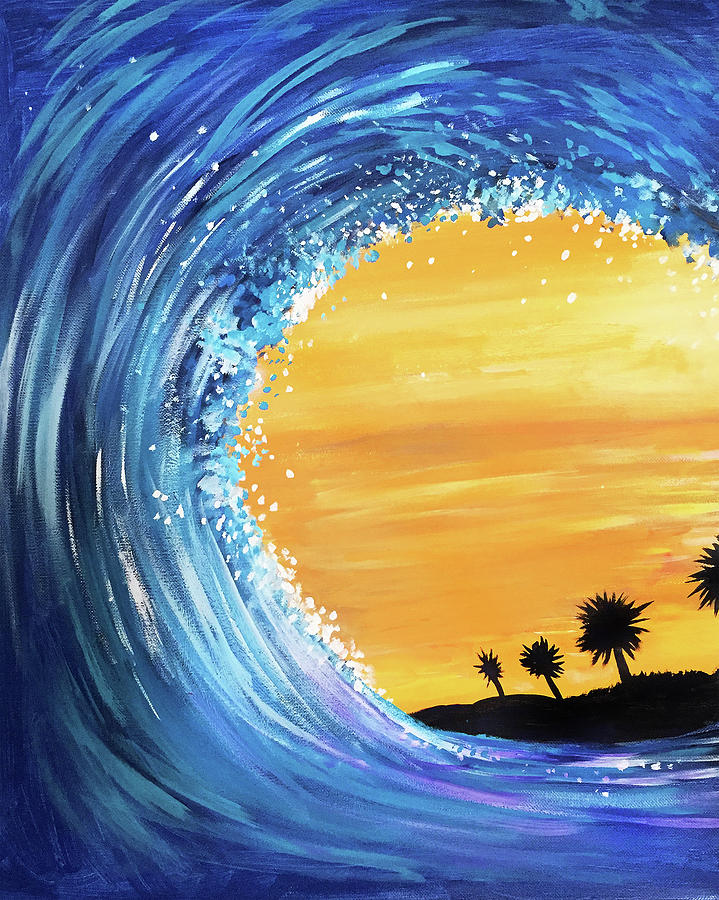The image is a visually striking painting depicting a powerful ocean wave dominated by shades of blue and white. The wave takes the form of a large, curling C-shape that stretches from the bottom right corner, sweeping across the canvas to the bottom left corner, and then up towards the top right, creating a dynamic sense of motion as it begins to crash back down into itself. The background reveals a warm orange sky, suggesting a sunset or sunrise, adding a vivid contrast against the cooler tones of the wave. Silhouetted against this radiant backdrop are four black-shaded palm trees and a hillside or shoreline, giving the scene a tranquil, tropical feel as if one were gazing at a serene island landscape. The wave, meticulously created with swirling patterns, encircles the calm scenery tucked within its embrace, showcasing the artist's skill in blending movement and stillness.